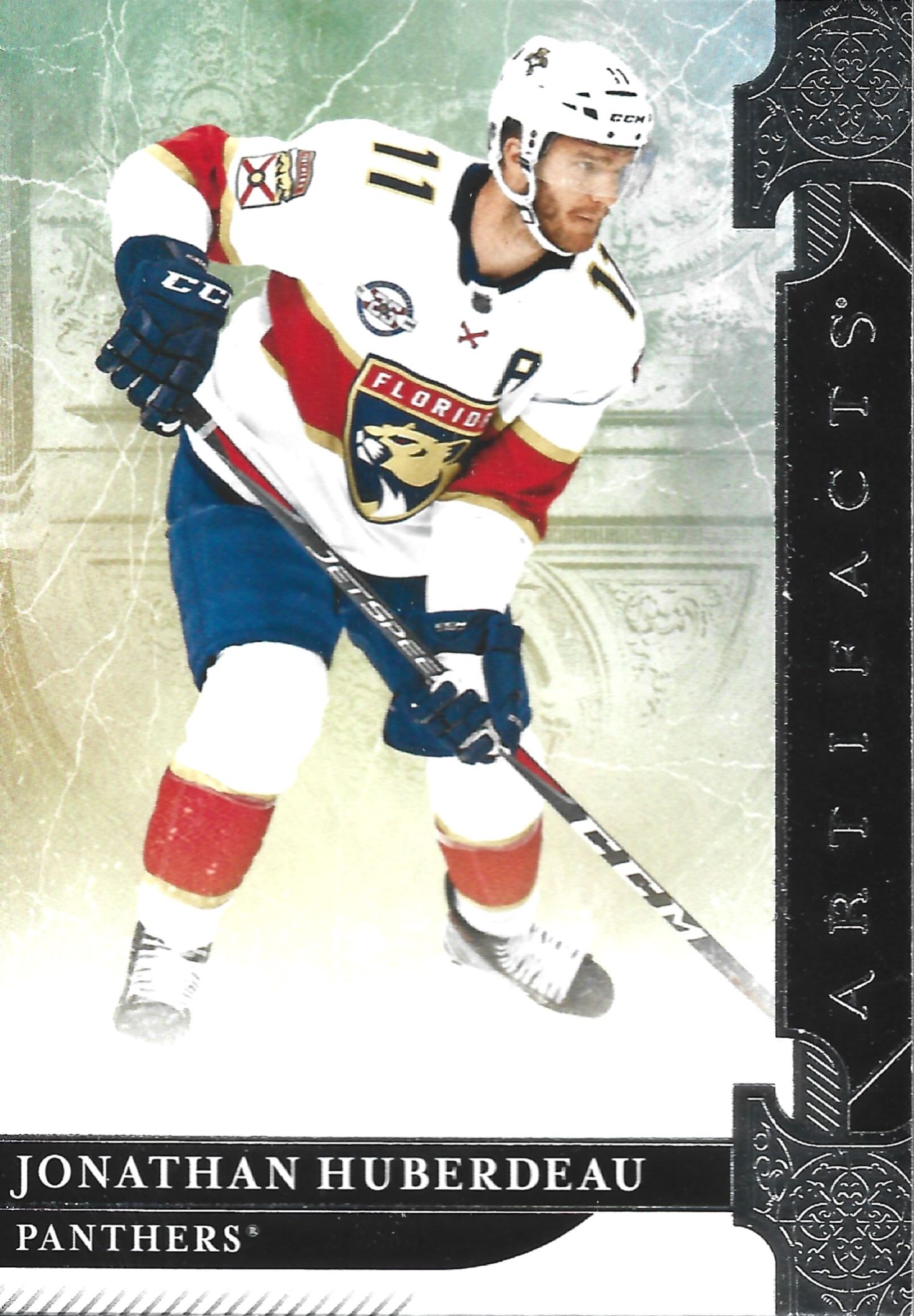The image features a Florida Panthers hockey player, Jonathan Huberdeau, captured in a vertical color photograph, likely from a sports trading card. Huberdeau is centered in the image, donning a white jersey accented with red and gold, and blue gloves. His uniform includes distinctive white, blue, and red pants, complemented by black skates with white laces. A white helmet adds to his gear as he holds a black hockey stick, marked with white "CCM" text, positioned towards the bottom right of the frame.

Along the bottom of the image, in white text on a black background, his name "Jonathan Huberdeau" is displayed with "Panthers" written below it in slightly smaller text. A black border surrounds the photo featuring decorative white elements at the top and bottom, and on the right side, the word "Artifacts" is inscribed in white. The Florida Panthers’ Wildcat logo, shaped like a shield with the letter "A" in black text, is visible on his uniform, highlighting his team affiliation. The setting suggests a pre-game introduction on the ice, capturing a poised and ready-to-play Huberdeau.